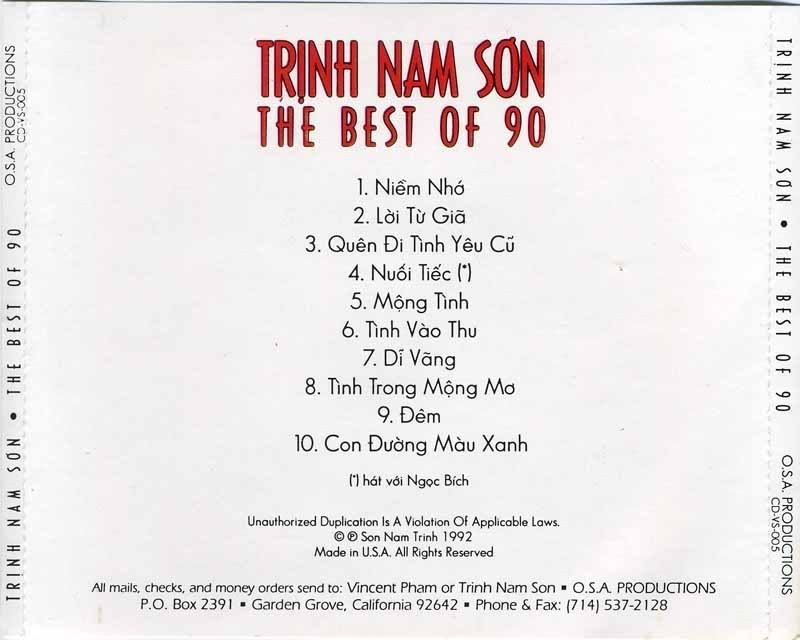The back cover of the CD album, nestled between the outer plastic casing and the CD holder, is predominantly white with mirrored periphery text on thin perforated strips. The text on the strips lists the album title and producer, reading "Trinh Nam Son, The Best of 90, OSA Productions CD VS005," replicated on both the left and right sides descending from the top.

At the top center, the title "Trinh Nam Son, The Best of 90" is prominently featured in dark red font. Below this, the tracklist from 1 to 10 outlines the songs, all in Vietnamese. The tracks are: 1. Niamh Non, 2. Loi Tu Gai, 3. Queen Dai Tin Ye Tu, 4. Noi Tai, 5. Mong Tin, 6. Tin Vao Dur, 7. Dai Quang, 8. Tin Trong Mong Mo, 9. Dem, 10. Cong Duong Mau Zong.

Toward the bottom, contact details are provided for correspondence. It reads, "All mails, checks, and money orders send to Vincent Pom or Trinh Nam Son at P.O. Box 2391 Garden Grove, California 92642," along with the phone and fax numbers, suggesting that OSA Productions is based in the United States.